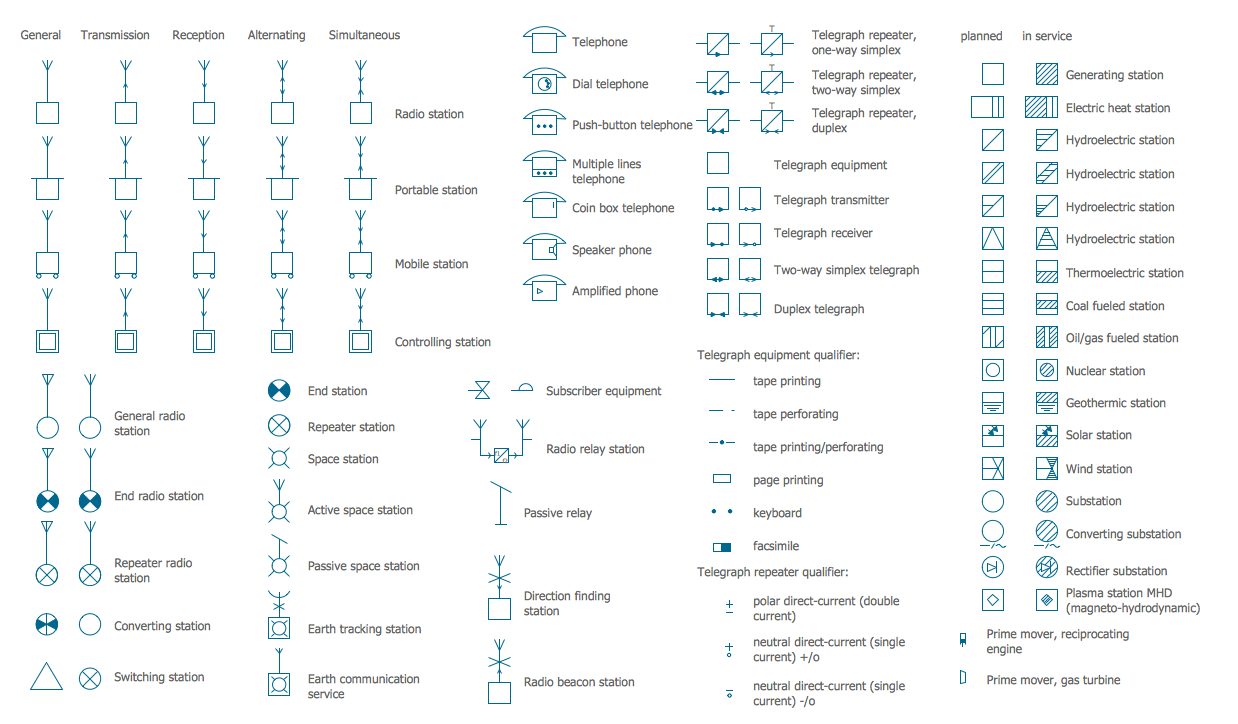The image is a highly detailed diagram serving as a map legend that provides information about various types of utility and telecommunications stations, as well as their planned locations. It identifies general radio stations, repeater radio stations, converting stations, and switching stations. Additionally, it includes icons representing different telecommunication methods such as telephones and telegraphs, as well as various power sources such as electric heat stations, hydroelectric stations, coal fuel stations, and oil gas stations. The diagram is characterized by its use of black font for text and light blue and dark blue colors for the icons and other diagram portions, presenting a comprehensive overview for what appears to be a planning committee involved in communication and energy infrastructure.